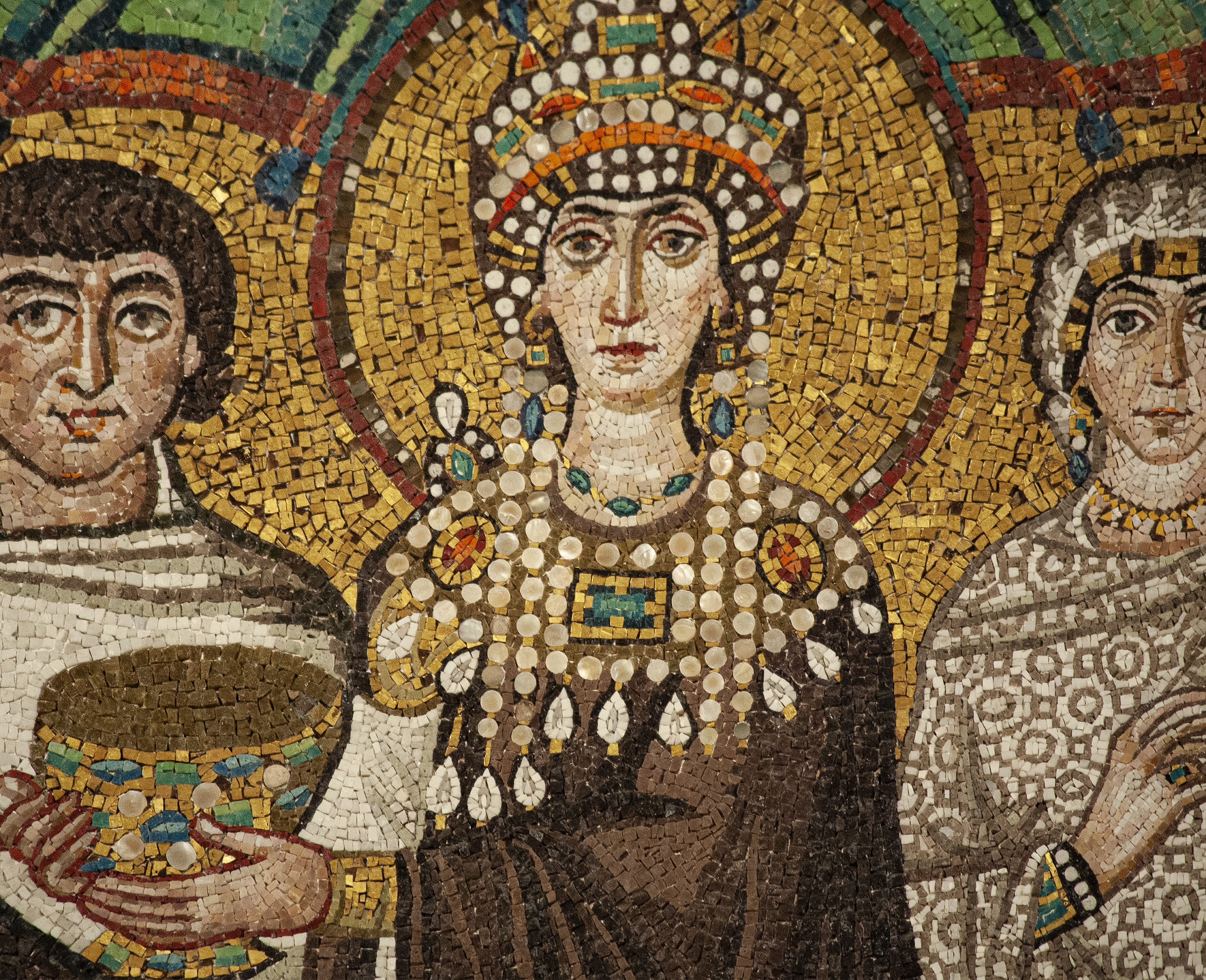The image showcases an impressive Byzantine-era mosaic featuring three distinct religious figures arranged side by side. The intricate mosaic is composed of numerous colored stones meticulously placed to create a detailed and vibrant scene. 

On the left is a man with dark brown hair and brown eyes, garbed in a white toga, who appears to be holding a chalice or a cup. This male figure gazes directly at the observer, adding an engaging element to the scene. In the center stands a woman adorned with an elaborate headdress, rich in beads or large pearl-like ornaments, cascading down and covering parts of her ornate brown robe. She is also holding a chalice encrusted with blue, green, and white jewels, emphasizing the mosaic’s attention to intricate details. 

The rightmost figure is clad in a geometric-patterned brown and white robe, complemented by a matching headdress. This person, possibly with braided white hair, wears a white bracelet and a blue ring. The background features golden circles outlined in red, with touches of green, adding to the divine and regal aura of the scene.

Overall, this mosaic is a testament to meticulous craftsmanship, reflecting the rich cultural and religious tapestry of the Byzantine era. Each stone, carefully placed, contributes to the grandeur and complexity that words alone struggle to capture.